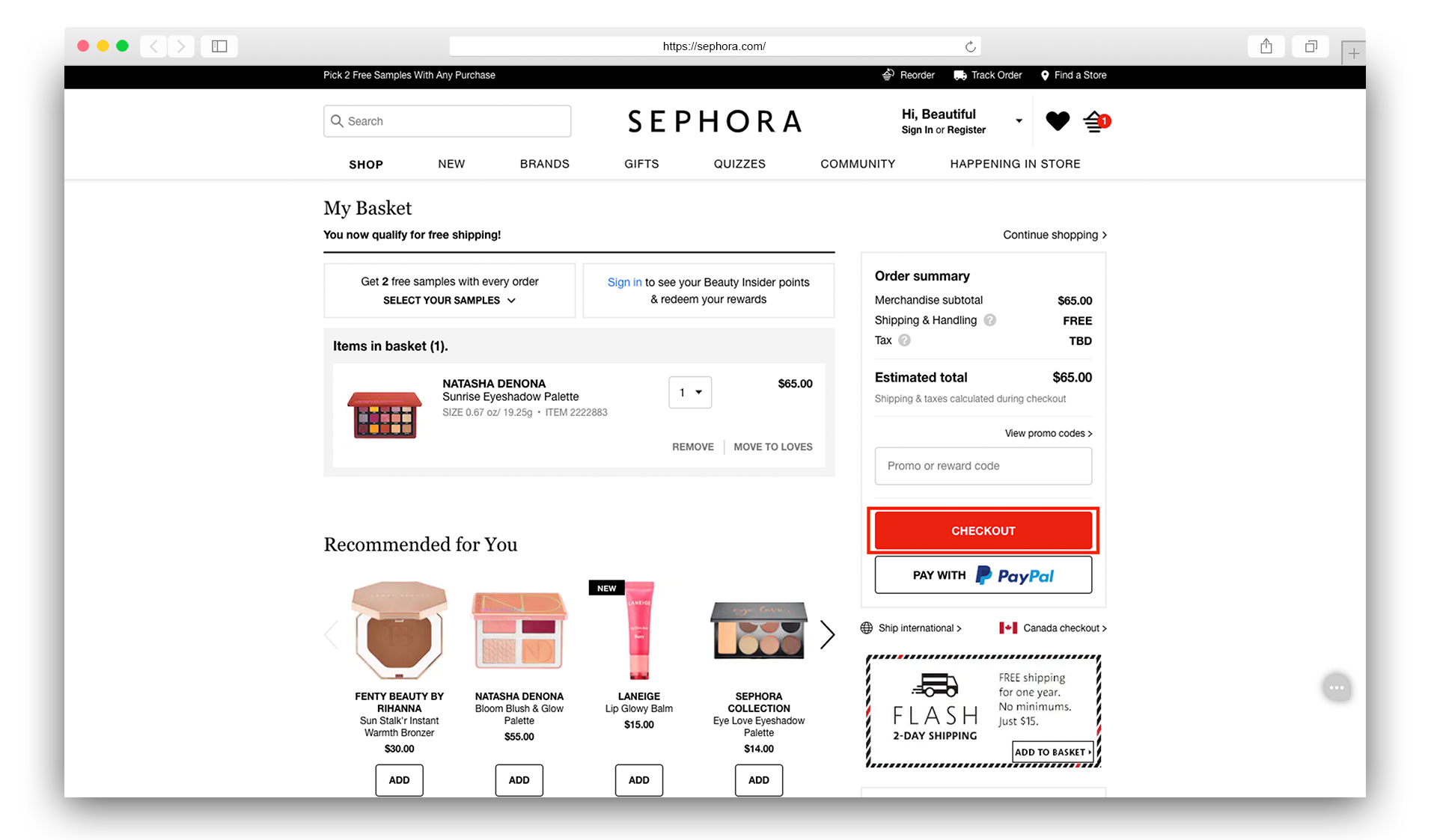Here is a cleaned-up and detailed caption for the image description:

---

The landing page of Sephora, viewed through a Safari browser, presents a sleek and user-friendly interface. At the top center, "Sephora" is prominently displayed as the title. On the left side of the title is a search bar, while the right side features a Sign In or Register section, a black heart icon indicating favorites, and a shopping cart displaying a red notification badge with the number one. Below the title, there are several navigation tabs arranged in a row: Shop, News, Brands, Gifts, Quizzes, Community, and Happening in Store.

Immediately below these tabs, users can find the My Basket section. Currently, the basket contains a Natasha Denona Sunrise eyeshadow palette, characterized by its pink hue and collection of 15 distinct shades. The palette is listed with a quantity of one at a price of $65, with an item number 2222883.

The section beneath the basket is titled "Recommended For You," showcasing four items. The first item on the left is a warm bronzer compact makeup from Fenty Beauty by Rihanna. The second item is another product from Natasha Denona, a compact featuring four color palettes in a square container marked with the initials "ND," priced at $55. The third product, labeled "sixth," is a Laneige Glowy Lip Balm, noted for its pink color. Another "sixth" item is an eyeshadow palette consisting of six shades, one of which appears suitable for cheek application rather than eyeshadow. Each product in this section includes a prominent "Add" button below it for easy addition to the basket.

To the right of these sections is the Order Summary box, detailing the current purchase. The list includes a Merchandise Subtotal of $65 and free Shipping and Handling, with Taxes to be announced. The Estimated Total also stands at $65. Below these details is a Promo or Rewards code bar and a red Checkout button, complemented by a Pay with PayPal button for alternative payment options.

A banner in the bottom right corner advertises a special offer: Flash 2-Day Shipping for Internet purchases, providing free shipping for one year with no minimum order requirement for just $15.

---

This detailed caption accurately describes all the elements on the Sephora landing page, ensuring clarity and coherence.